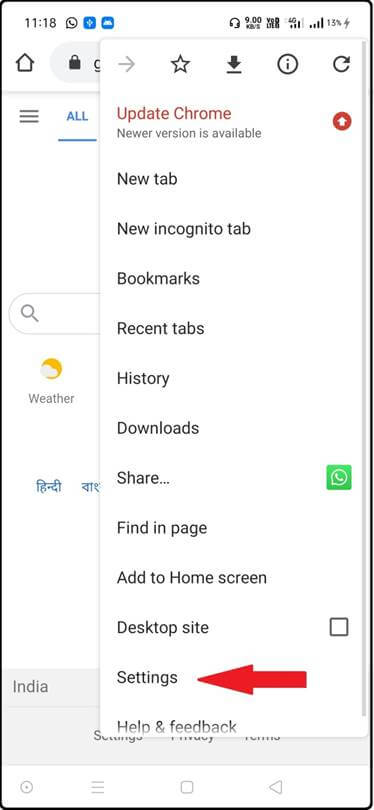This image is a detailed screenshot of a mobile website viewed in the Google Chrome browser. A drop-down menu dominates the screen, obscuring most of the main page beneath it. The menu, featuring a white background with black text, highlights the "Update Chrome" option in red, indicating that a newer version is available. 

The menu includes several options listed sequentially: 
- Update Chrome (selected)
- New Tab
- New Incognito Tab
- Bookmarks
- Recent Tabs
- History
- Downloads
- Share (accompanied by a small Google Voice icon)
- Find In Page
- Add to Home Screen
- Desktop Site (with an unchecked checkbox beside it)
- Settings (marked by a prominent red arrow)
- Help and Feedback

Visible at the very bottom, partially hidden by the drop-down menu, is a Google Search page displaying the current weather conditions.